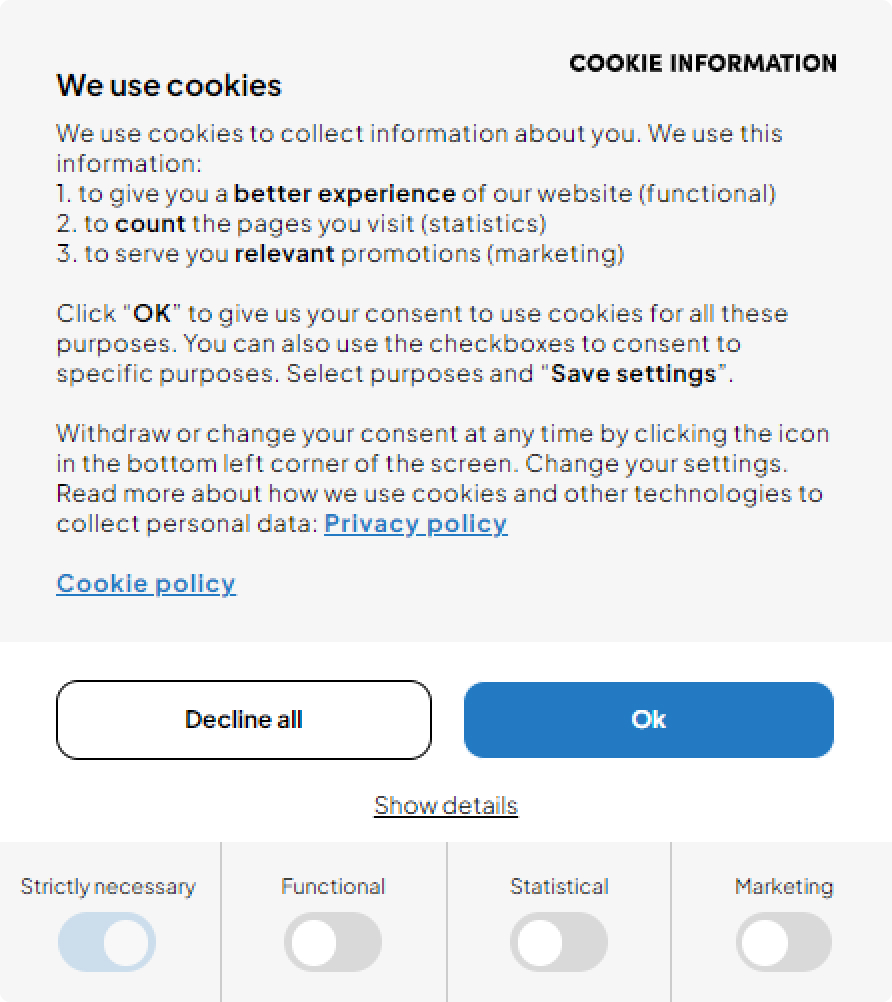The image depicts a detailed website cookie consent form against a gray background, featuring comprehensive information and user interaction options presented in black text. The form outlines that cookies are used to collect information about visitors, aimed at providing an enhanced user experience, tracking page visit statistics, and tailoring relevant marketing promotions. 

Users are given the option to click "OK" to consent to the use of cookies for these purposes, or customize their consent through checkboxes for specific purposes such as personal data, privacy policy, and cookie policy. A notable feature on the form is an icon in the bottom corner of the screen, allowing users to withdraw or change their consent at any time.

The interactive elements include a prominent “Decline All” button in a rectangular format at the bottom, alongside a blue “OK” button. Additionally, there is a gray "Show Details" button, underlined for emphasis, which expands to reveal further cookie policy details. The form categorizes the cookie options into "Strictly Necessary," "Functional," "Statistical," and "Marketing," providing users with clear and concise options for their cookie preferences.